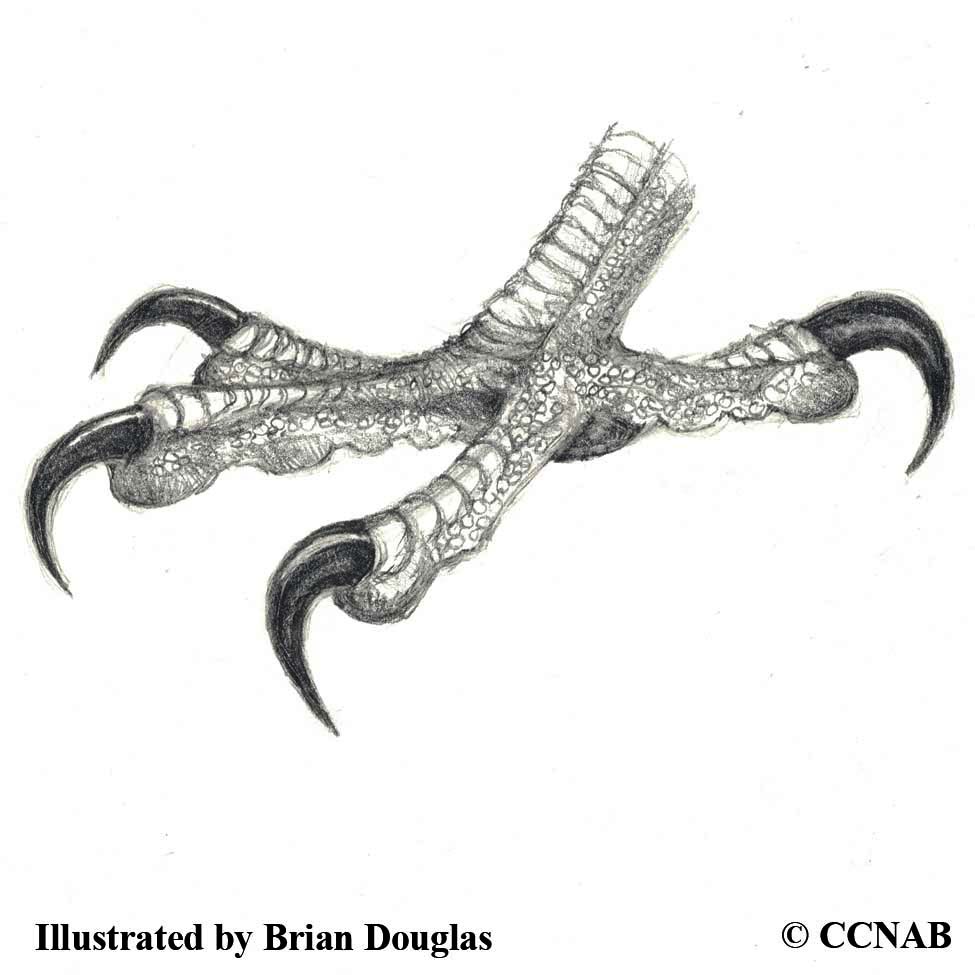This black and white sketch, rendered in ink or pencil, depicts the detailed claw of a bird, specifically noting the intricate structure of a chicken's foot. The claw features four talons—three extending forward and one positioned in the back—all adorned with sharp, curved black hooks and textured with scaly patterns. The toes, thin and spiny, are meticulously shaded and display outlined circles that enhance the reptilian appearance. The leg stops just above the foot, giving a cropped effect. At the bottom left corner, the illustration is boldly credited with "Illustrated by Brian Douglas," accompanied by a copyright symbol and the initials "CCNAB" on a plain white background.